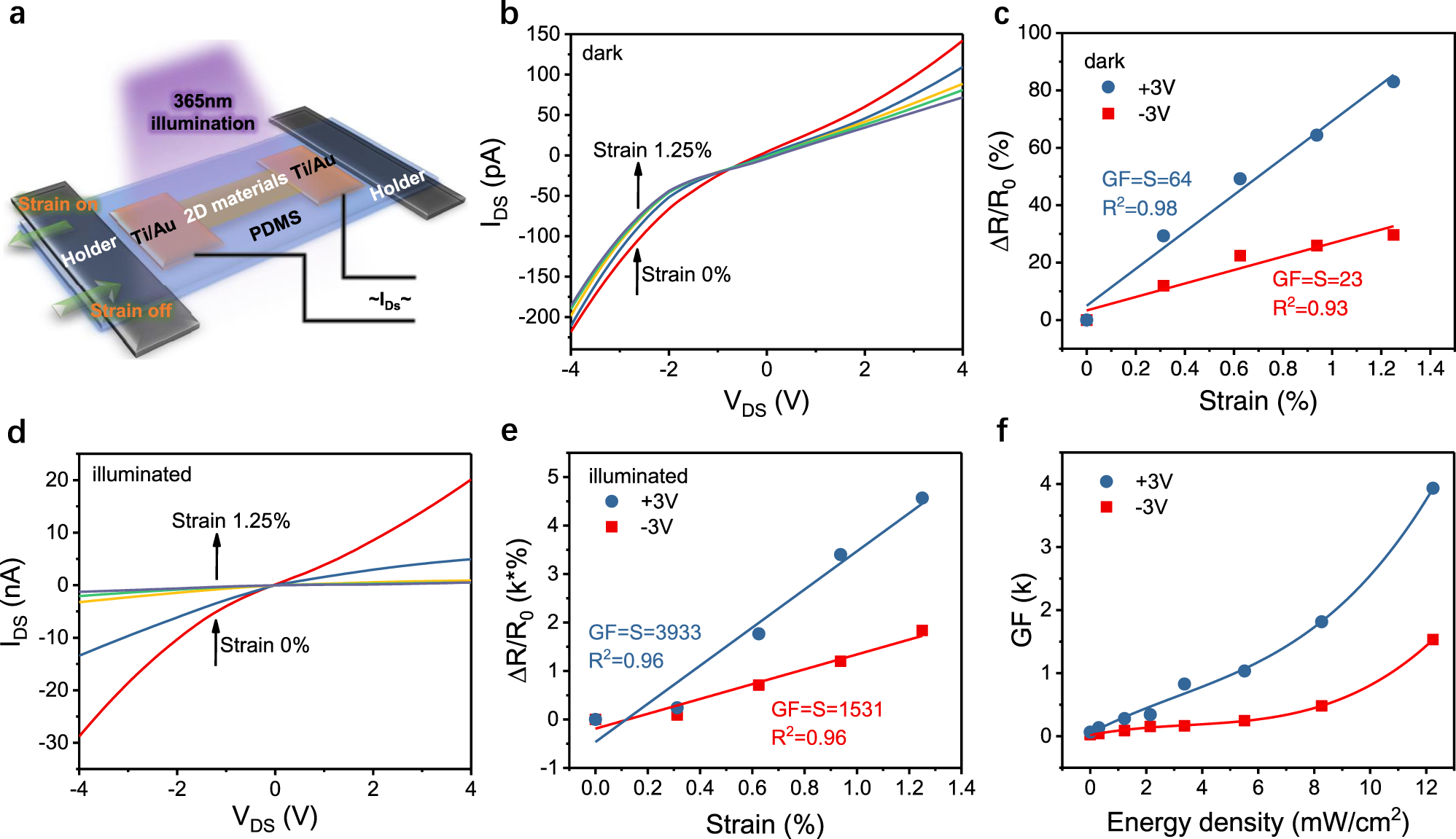This detailed caption describes a series of labeled infographics or graphs, each with its own specific set of data and annotations:

---
**Figure A:** This infographic, located in the upper left corner, features a color-coded image with blue, purple, and brown tones. The title "2D Materials" is prominently displayed with the labels "TI/AU" on both sides. Below the image, the acronym "PVMS" is noted. A gray strip on the right side reads "Holder," and in purple text, "365 NM Illumination" is highlighted. On the left side, another gray strip labeled "Holder" includes arrows; the arrow pointing left is marked "Strain On," while the arrow pointing right says "Strain Off."

**Figure B:** The upper part of this graph lists data for "IDSPA" from -200 to 150 in increments of 50. The "VDSV" values range from -4 to 4 in increments of 2.

**Figure C:** This graphic displays "R/R%" with values ranging from 0 to 100% in increments of 20%. "Strain" is measured from 0 to 1.4 in steps of 0.2.

**Figure D:** The vertical axis for this chart represents "IDSNA" with values from -30 to 20 in increments of 10. The horizontal axis shows "VDSV" ranging from -4 to 4 in increments of 2.

**Figure E:** The y-axis in this graph is labeled "R/R (K%)" with values from -1 to 5 in increments of 1. The x-axis tracks "Strain" from 0 to 1.4 in 0.2 increments.

**Figure F:** This last infographic details "GF (K)" with values from 0 to 4 in steps of 1 on the y-axis. Additionally, "Energy Density (W/MW/cm²)" ranges from 0 to 12, increasing by 2. The graph features blue and red line plots indicating specific data points.

---
This caption offers a thorough breakdown of the informational content and layout present in each infographic.